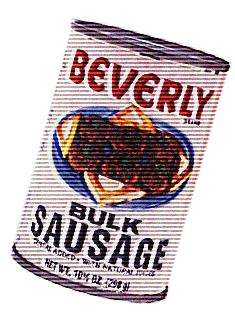This is a pixelated graphic of a tin can set against a pure white or transparent background. The tin can is viewed from the front, prominently displaying a white label. At the top of the label, the word "Beverly" is written in bold red letters. Just below "Beverly," slightly to the right, there is smaller, unreadable text. Below this, there's an illustrated graphic showing a blue plate with a brown item on it. Under the illustration, the label reads "Bulk Sausage" in blue font. Further down the label, there's another section of small, unreadable text followed by the can's weight, which is also indiscernible due to the pixelation.